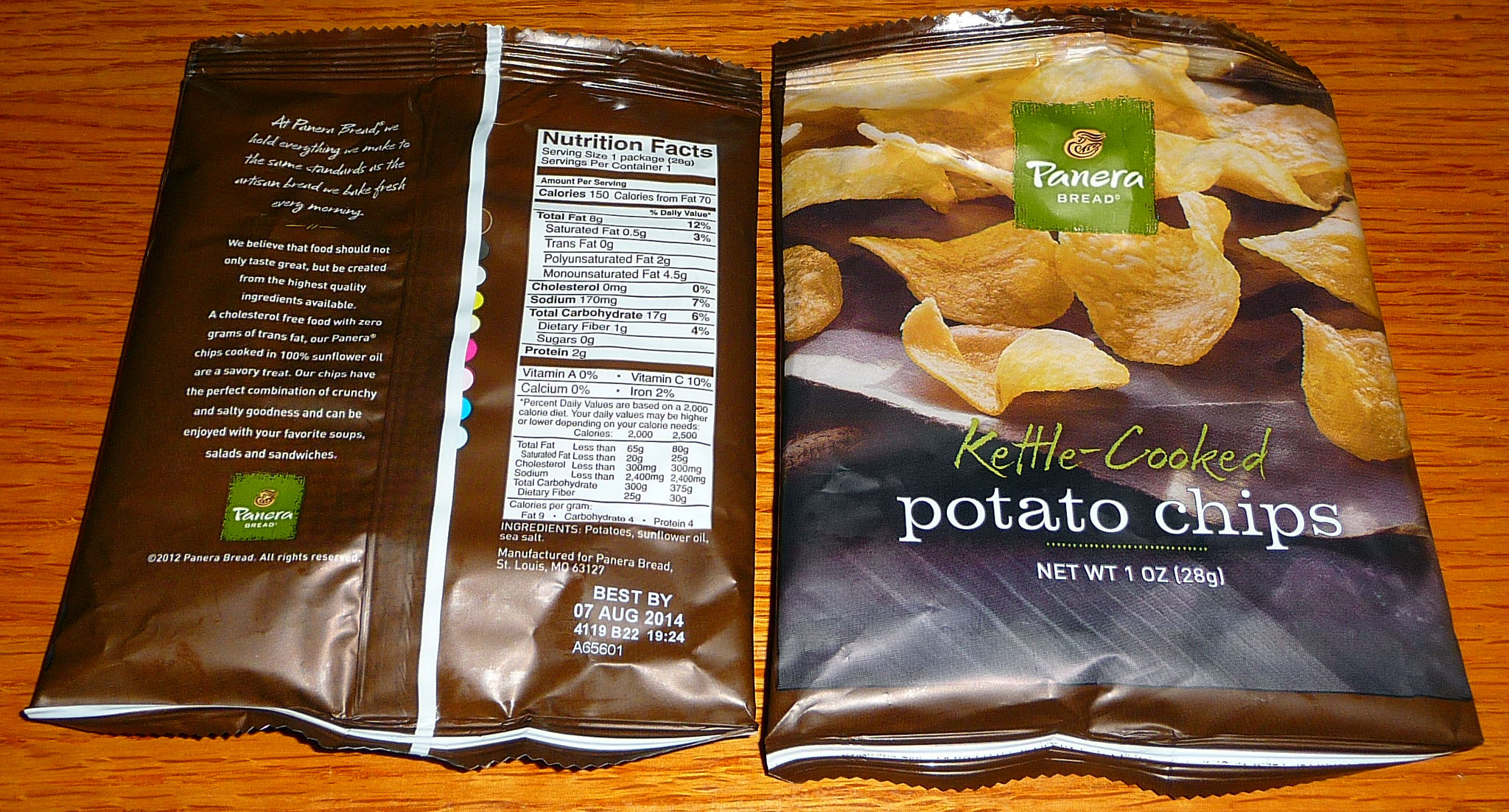A round table is in focus, with two black bags positioned prominently at either side. The bag on the left features a distinct line running through its center. To the right, a bag placed in the foreground contains a variety of items, including a pack of chips. The chips bag sports green lettering that reads "Kettle-Cooked Potato Chips" and includes additional details such as "net weight one ounce (28 grams)." The packaging features a visible green square emblem with "Panera Bread" inscribed on it. Below the text, there are white lights and a black line, possibly part of the design. To the left of the table, several signed shirts displaying the Panera logo are noticeable. Each shirt bears the inscription “best bought: 07 August 2014.”